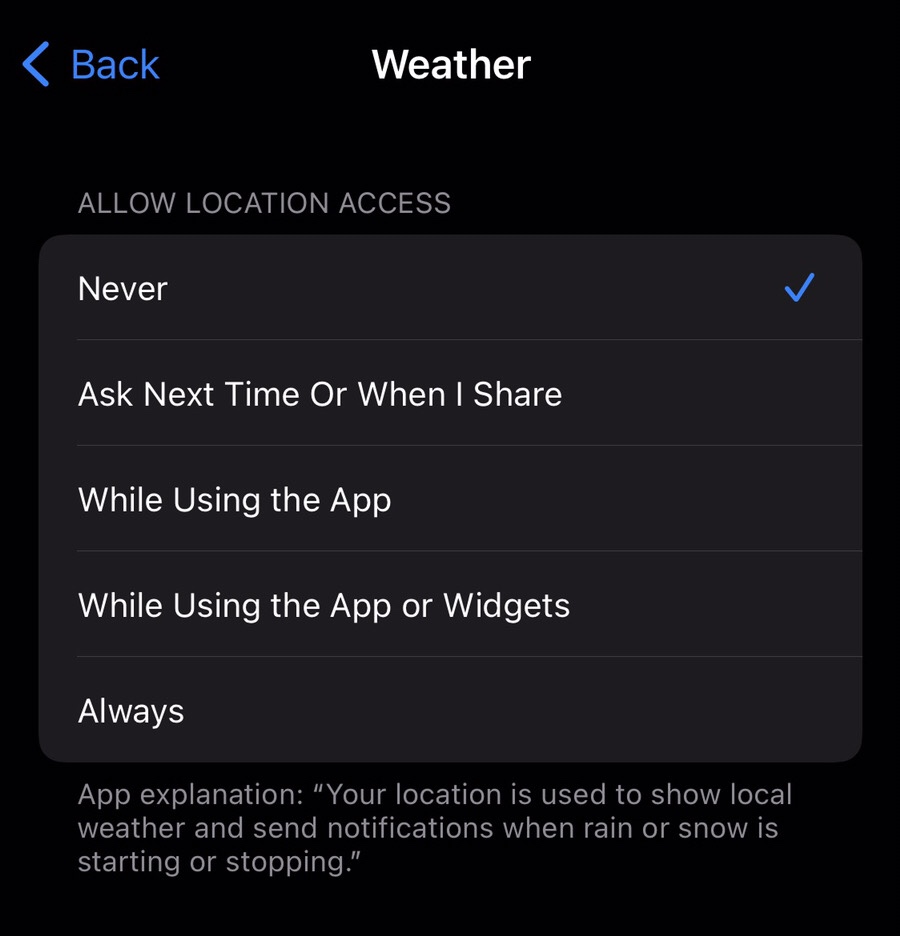This screenshot features an all-black background, predominantly showcasing location access options for a weather application. In the top left corner, there's a blue "Back" button accompanied by a left-pointing caret symbol. On the right side of the screen, centered horizontally, the word "Weather" is displayed in white text. Directly below it, the phrase "Allow Location Access" appears in light gray letters.

Beneath this, a medium-gray box is segmented into five options for location access permissions, each labeled in white text. The first option, "Never," is selected, indicated by a blue checkmark to the right. The second option, "Ask Next Time Or When I Share," is not highlighted and does not have a checkmark. Following this, the third and fourth options are "While Using the App" and "While Using the App or Widgets," respectively. The final option is "Always."

At the bottom of the options list, there's a section labeled "App Explanation" containing a brief description in quotes: "Your location is used to show local weather and send notifications when rain or snow is starting or stopping."

The image lacks any contextual markers to indicate whether it was taken from a phone, laptop, or another type of device.